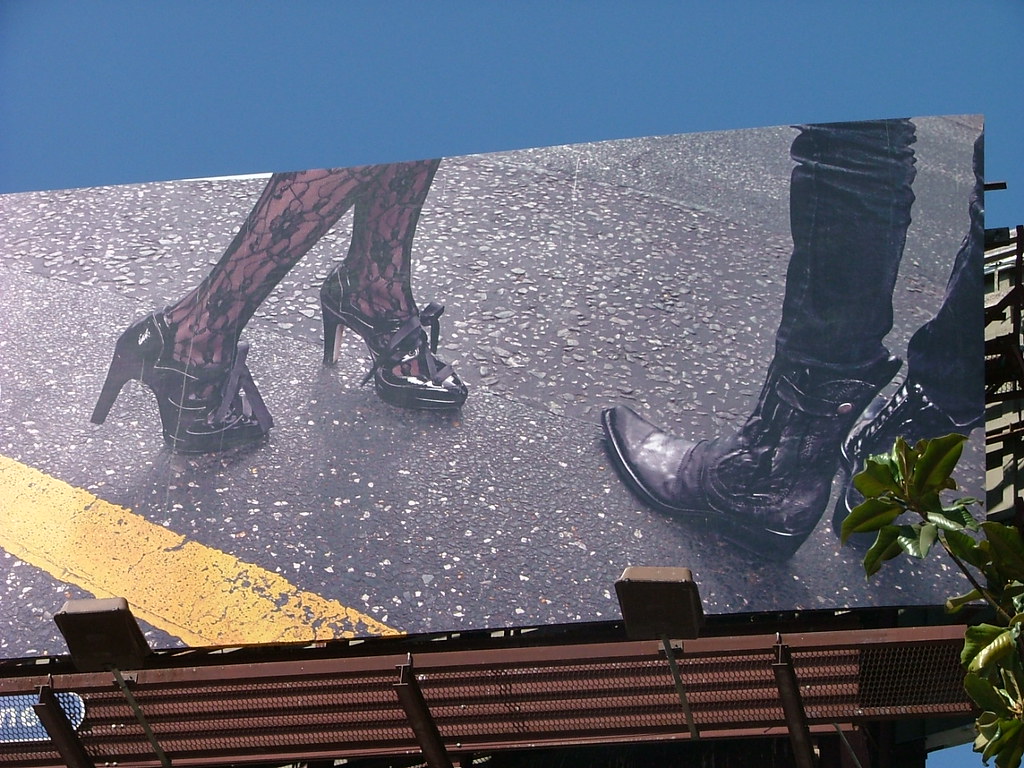In this vivid, color photograph, a billboard prominently stands against a backdrop of clear blue sky, capturing the essence of urban life. The billboard itself depicts a city street with a yellow line stretching diagonally towards the left edge, guiding the viewer's eye through the scene. On the left side of the billboard, a pair of elegant legs, likely female, clad in black lace stockings and stylish high heels laced up with black ribbons, add a touch of sophistication. The right leg is poised behind the left with the foot gently lifted off the ground, suggesting movement. To the right of this billboard image, another pair of legs appears, dressed in dark blue jeans and adorned with sharp, black cowboy boots featuring pointed toes, providing a contrasting, rugged aesthetic.

Adjacent to the billboard, a building looms just behind it, adding depth and context to the urban setting. In the bottom right corner of the overall image, a tall green leafy tree or plant adds a hint of nature, softening the otherwise bustling city scene. This image is strikingly detailed, capturing an intriguing juxtaposition of fashion and everyday life, all without a single word on the billboard.